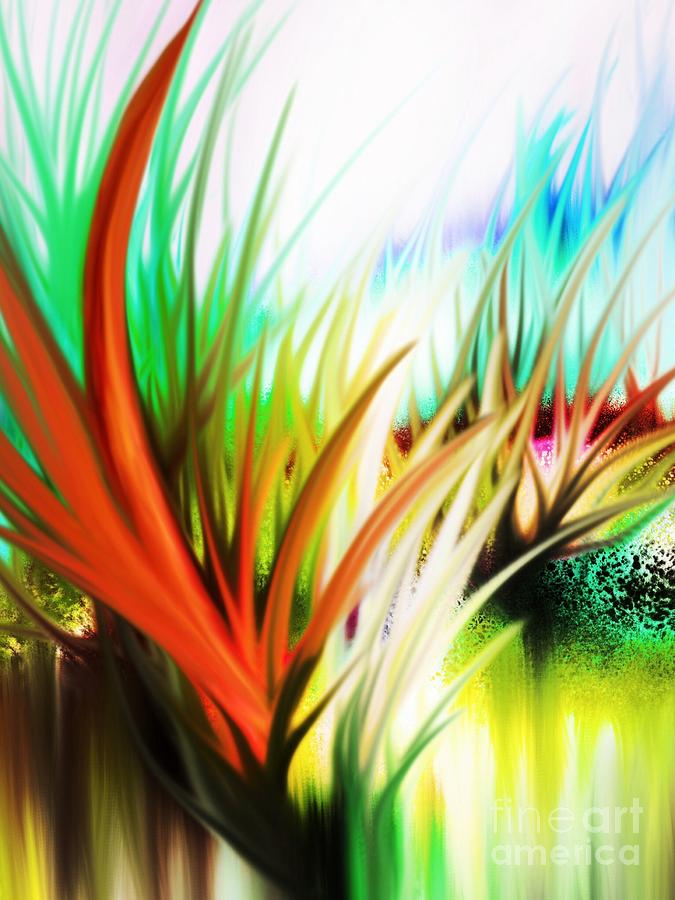This digital artwork features a mesmerizing, abstract depiction of grasses with a rich, psychedelic palette. At the center-left, a prominent pair of grass blades starts green and transitions to red as they extend leftward. Surrounding these blades, additional strands of grass shift through vivid yellows and greens. To the right, grasses display a dynamic color gradient between red, yellow, and green. Further back, blue and purple hues emerge, adding depth to the composition. The background sky is a stark white, contrasting with the colorful grasses. The bottom third of the image features streaks of yellow, green, and black, suggesting a water body or marshland. In the bottom right corner, a semi-transparent white watermark reads "Fine Art America," indicating the artwork's origin. This depiction combines traditional grass motifs with artistic techniques, likely digital, enhancing the overall visual impact with its vibrant colors and flowing line art.